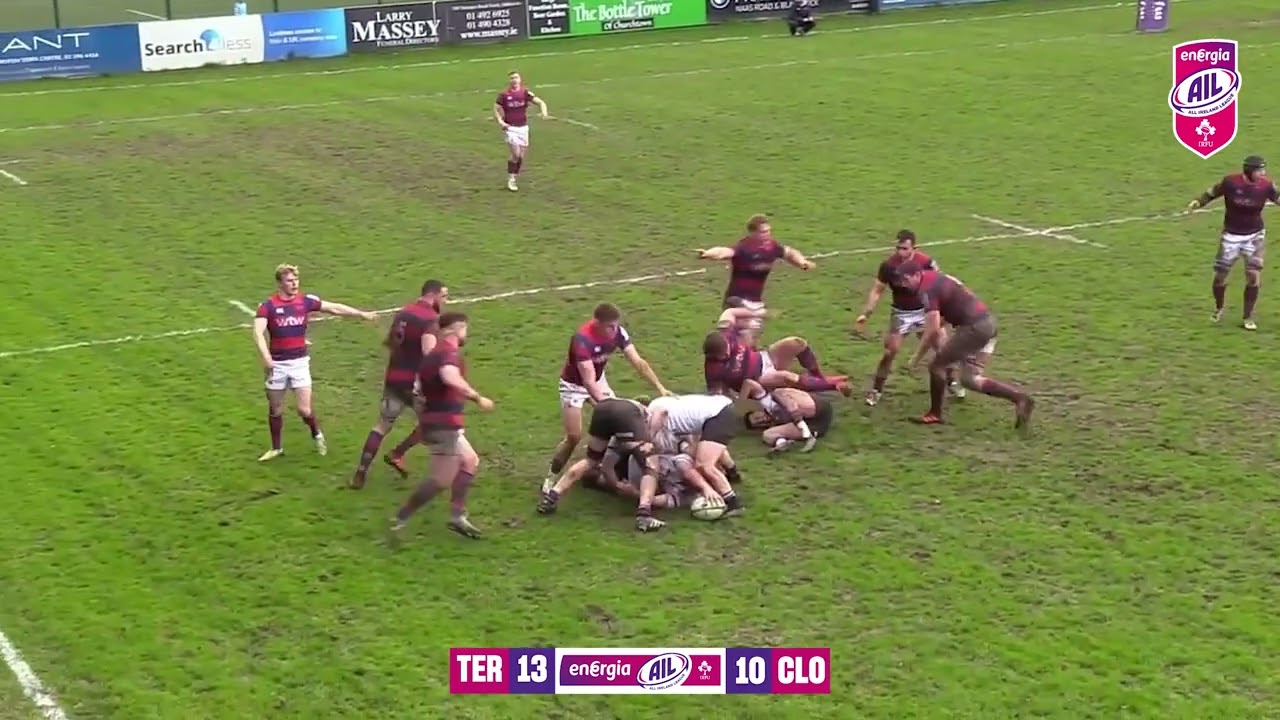This image is a detailed, overhead drone photograph of a rugby match taking place on a muddy, grassy field that shows signs of recent rain, with green patches interspersed with brown. The main focus is on several players engaged in a physical tussle in the center of the field; some are on top of each other, covered in mud, while others are aggressively blocking or running. One team is wearing red shirts with dark blue stripes and white shorts, while the opposing team is in white jerseys with black shorts. The scene suggests a brawl or intense physical play. In the background, there are barricades adorned with various sponsor advertisements. A digital scoreboard at the bottom center of the image indicates the teams and their scores: T.E.R. with 13 points on the left and C.L.O. with 10 points on the right. The photograph is in landscape orientation, emphasizing the realistic and chaotic nature of the sporting event.